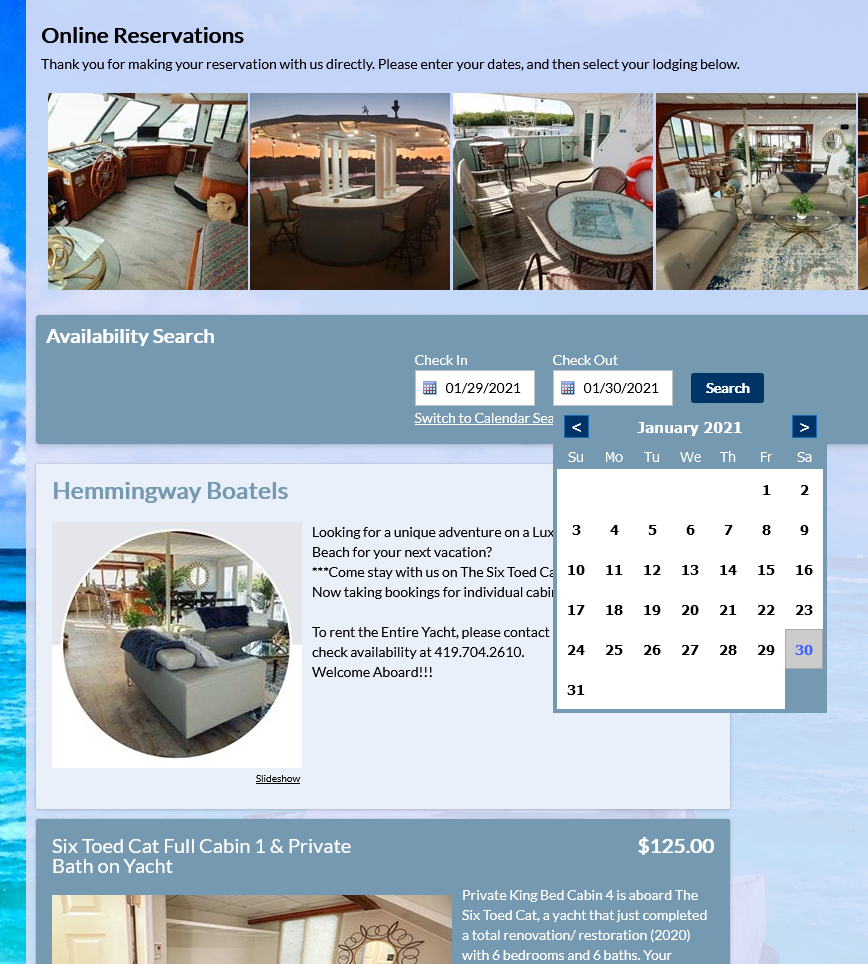A screenshot of an online reservation interface on a Windows system. The vertical screenshot displays a portion of the Windows background on the left, indicating it's a Windows operating system. The main section of the screenshot showcases an online reservation page with a light blue background. At the top, it reads "Online Reservation" followed by a thank you message: "Thank you for making your reservation with us directly." Below this, users are prompted to "Enter your date, select your lodging below."

Next, four images of different lodging options are lined up side by side. Beneath these images, a darker blue banner contains the text "Availability Search" on the left side. To the right, a section allows users to input their check-in and checkout dates with a search button following. The dropdown calendar for the checkout date is active, displaying January 2021, with the 30th highlighted.

Directly below this, there is information about available lodgings. The first listing, partially obscured by the active dropdown calendar, shows "Hemingway Botels" with an image of the lodging. Nearby, another listing under a darker blue header reads "Sick Toad Cat," featuring "Full Cabin One" and "Private Bath on Yacht" for $125. The accompanying picture and text for this listing are slightly cut off due to the framing of the screenshot.